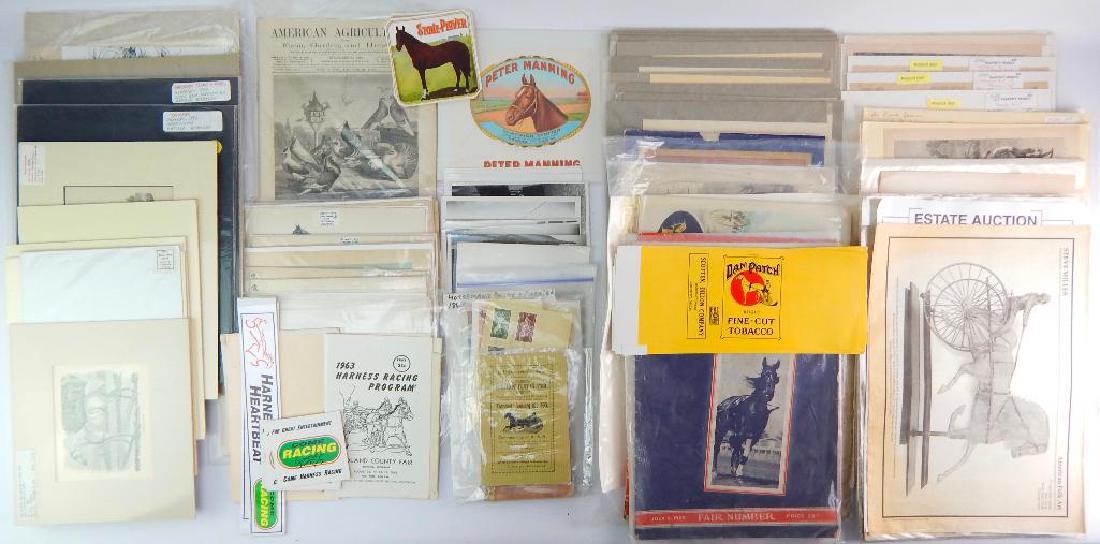The image depicts an overhead view of five neat columns of assorted cards, each resembling small documents or inserts that one might find in a wallet, some encased in plastic covers. The cards, placed atop a solid medium gray background, vary in size and content. The first column contains six or seven cards, predominantly light-colored with two darker ones. The second column features a mix of card sizes, including one with a top image of a horse. In the middle, the third column prominently displays a card with a horse picture at the top; several smaller cards beneath this are in transparent plastic. The fourth column is fronted by a card with a horse image, and behind it, only the tops of other cards are visible. The fifth column's foremost card reads "estate auction" and includes a depiction of a horse and cart, fitting the recurring equine theme. Notable text across the group includes "fine cut tobacco" associated with an image of a horse labeled "Dan Patch" and "Peter Manning," also accompanied by equine imagery. The setting, bright and clearly lit, emphasizes the clarity and detail of the documents.